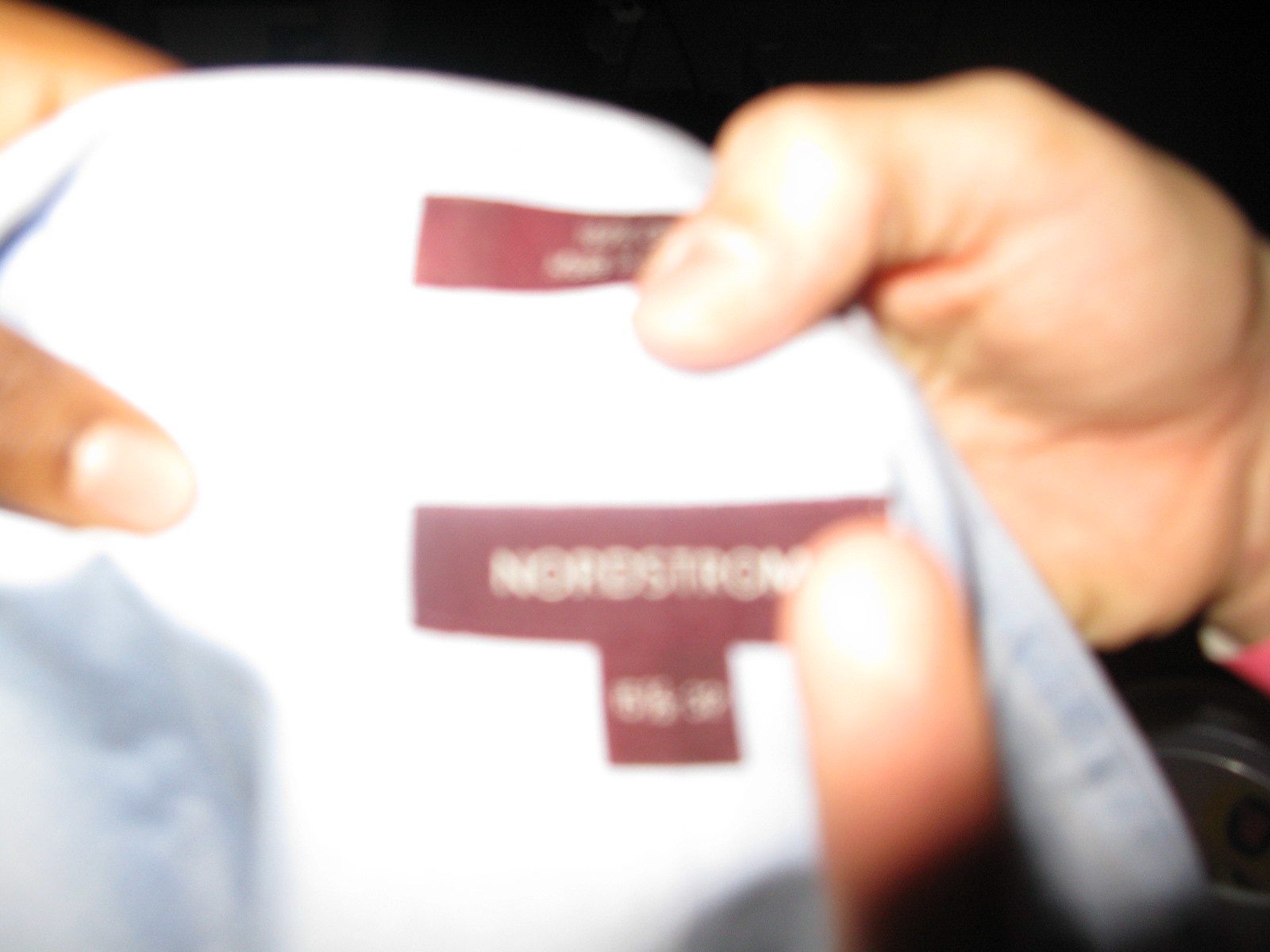This photograph captures an intimate, close-up moment of two distinct hands grasping a single object. The image is slightly blurry, obscuring fine details but revealing enough to create an intriguing scene. The hand on the right, with its inner palm facing the camera, is of a lighter skin tone, suggesting it belongs to one person, while the hand on the left, displaying only a finger and part of the nail, is of a darker skin tone, indicating a different individual. This juxtaposition supports the impression that two different people are involved. 

The object they are holding appears to be circular and made of a fabric-like material, possibly white, very light blue, or denim-colored. It features two red shapes that contain text, though the writing is too blurry to discern clearly. However, upon close inspection, a fragment of the text seems to read "Nordstrom" on the lower portion of the object. The dark, black background further isolates the hands and the object, emphasizing the interaction. The proximity of the hands and the way they cling to the object suggests a subtle tug-of-war, adding a layer of tension and intrigue to the scene.